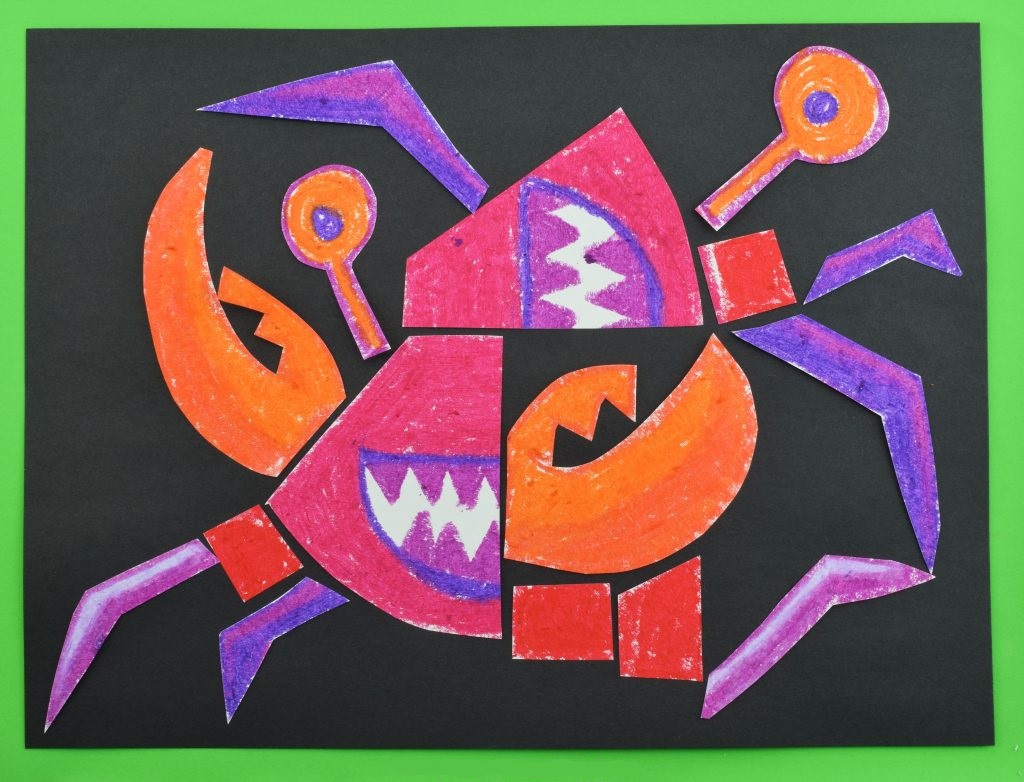This image features a vibrant piece of paper art displayed on a large sheet of black construction paper set against a green background. The artwork itself is an abstract, cubist-style depiction of a crab, rendered with crayon or wax pigment. The crab appears to be dissected and reassembled in a whimsical manner, resembling a stylized or child's interpretation of the creature. The crab's claws are colored orange, while its eye stalks are also orange with purple pupils. It has elongated purple legs and an expressive mouth featuring purple teeth, with a portion of the smile intriguingly bisected by the right claw. The detailed and colorful illustration stands out vividly against its contrasting background, creating a striking and imaginative visual piece.